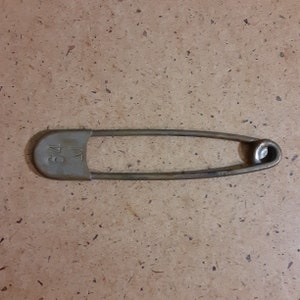This close-up image features an old-fashioned safety pin prominently displayed against a surface that resembles either a beige-ivory formica countertop or floor tile with gray and brown speckles. The pin, positioned sideways with the part that you push on to open it on the left, dominates the frame. It is made of sturdy, matted gray metal and shows signs of rust, suggesting its age. The pin is engraved with the number 64 at the top, which is an unusual characteristic, possibly indicating it may have been used for industrial purposes. Below the number, there is an arrow-like engraving and a coil at the bottom that holds the pin together when opened. This large, diaper-sized pin contrasts sharply with the marble-like pattern of the background, highlighting its robust and somewhat nostalgic design.